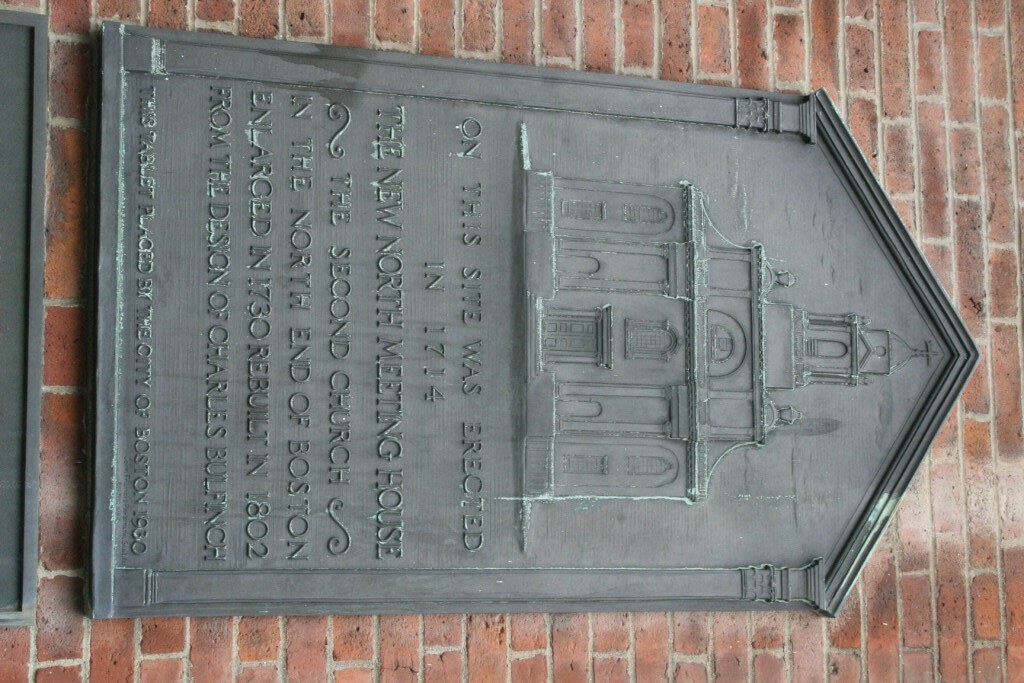This image depicts a historical marker plaque mounted on a red brick wall. The plaque, which appears gray, is shown sideways in the photo, making the text difficult to read without craning your neck. The marker is horizontally rectangular with a triangular edge on the right side. It has an engraved image of a three-story church that tapers into a triangular shape at the top, crowned with a tall pillar bearing a cross. The inscription on the plaque reads: "On this site was erected in 1714 the New North Meeting House, the second church in the north end of Boston, enlarged in 1730, rebuilt in 1802 from the design of Charles Bullfinch," although some portions of the text are illegible due to wear and the sideways orientation of the image.